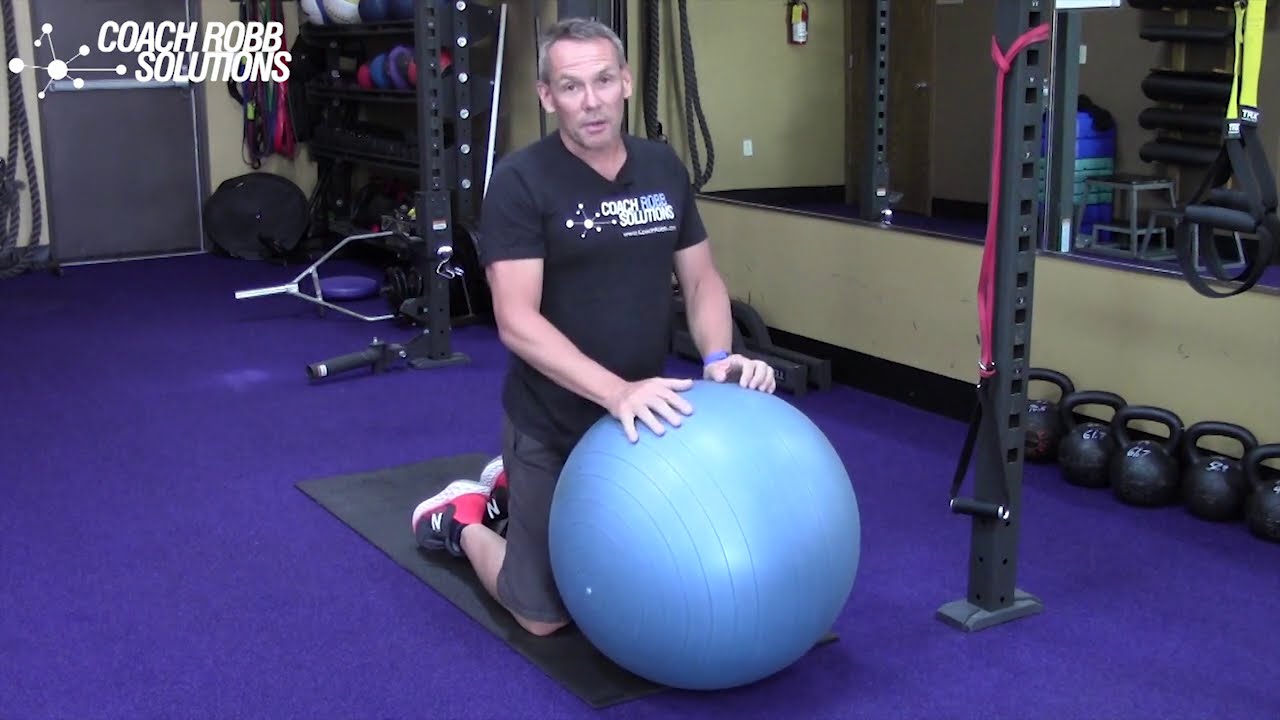This image appears to be an advertisement for "Coach Rob Solutions," prominently displayed in white text in the upper left corner, accompanied by a logo reminiscent of molecular structures—white circles connected by thin lines. The photograph is set in a gym with purple flooring, various weights, and a large mirror along the right-hand wall. In the center of the image, a man with short gray hair and fairly pale skin kneels on a black mat. He is wearing a black V-neck t-shirt that also reads "Coach Rob Solutions" with the same logo, and light gray shorts. The man is positioned behind a large blue stability ball, with both hands resting on it. He is also wearing red and black sneakers, likely New Balance, identifiable by the white "N" logos on the sides. Surrounding the man are gym equipment, including weights on shelves and a gray bar with a pulley mechanism, emphasizing the fitness setting.